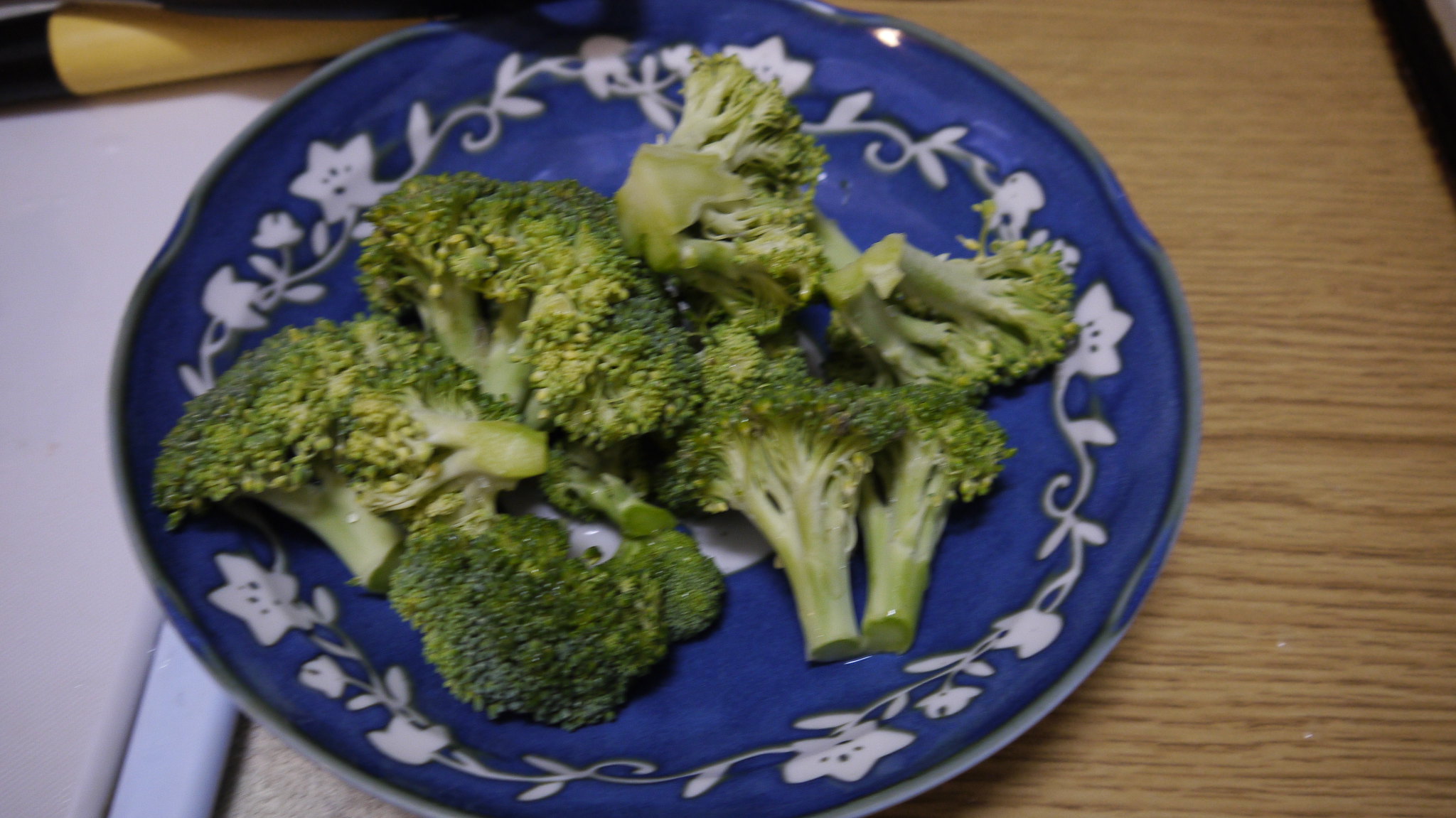The photograph is taken from above, angled slightly downward, capturing a light brown hardwood table. Atop the table, slightly to the left, there is a blue glass plate with a white floral design encircling its edges. The plate is filled with 5 to 8 pieces of broccoli, which range in color from dark green to a light green with hints of yellow, suggesting they may be cooked. The broccoli florets are arranged in a somewhat haphazard manner, occupying most of the plate. To the right of the plate, a pinkish dinner napkin is partially visible. The background reveals additional white and indistinguishable objects, possibly hinting at a countertop, with a vague yellow item blurred in the distance.